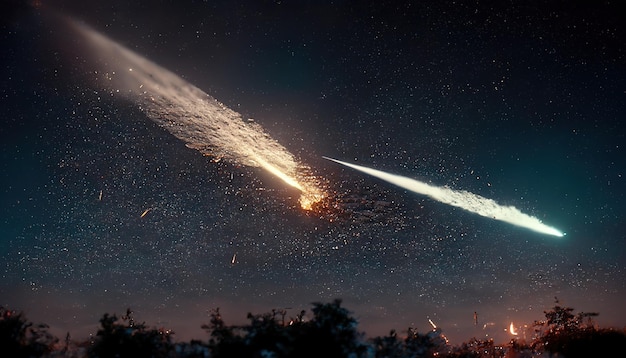The photograph captures a stunning night sky scene with two prominent comets and countless twinkling stars. The first comet, a brilliant blue-white streak, cuts across the bottom right corner of the image. The second comet, appearing larger and more vibrant with a fiery yellow hue, dramatically descends from the top left corner to the center of the frame. This larger comet leaves a trail of light and sparks behind it, giving a vivid sense of motion. The dark night sky features faint splashes of blue, and near the horizon, there is a hint of purple where the skyline meets the treetops. At the bottom of the image, the silhouette of a tree line adds a striking contrast to the luminous celestial display above.